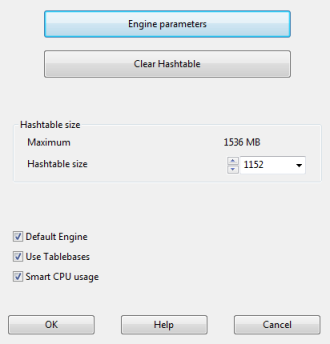This image appears to be a screenshot of a computer software dialog box with a light gray background and black text. At the top, there's a blue header labeled "Engine Parameters." Beneath this header is another labeled "Clear Hash Table." Central to the dialog box is a section titled "Hash Table Size," featuring two values: "Maximum," set to 1536 MB, and an adjustable "Hash Table Size," currently set at 1152 MB. On the lower left side, there are three options— "Default Engine," "Use Table Bases," and "Smart CPU Usage"—all marked with blue check marks. At the very bottom, there are three buttons labeled "Okay," "Help," and "Cancel" from left to right. The overall layout and styling suggest this is a digital interface likely related to software configuration or settings.